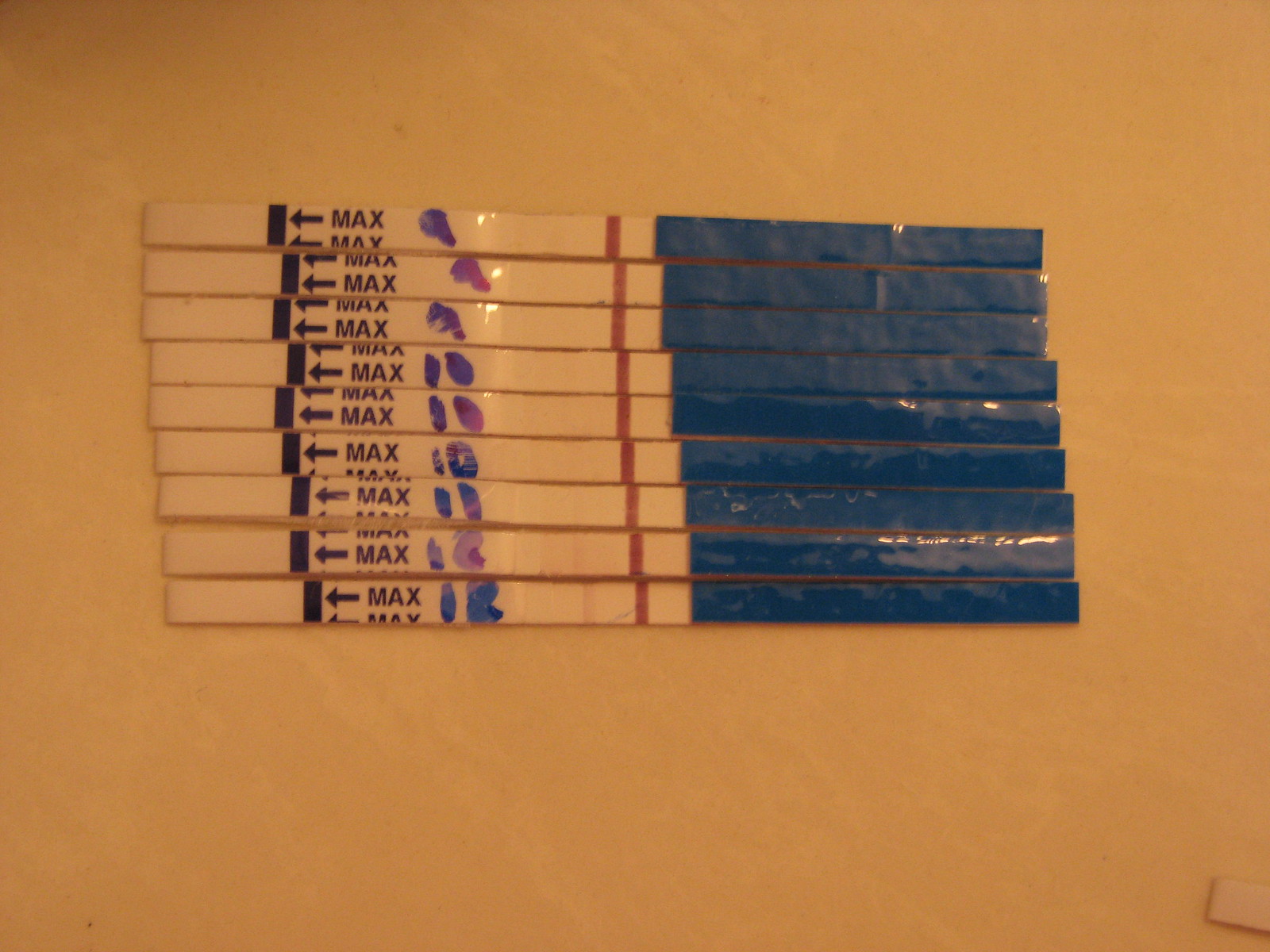The image showcases nine long, thin test strips meticulously aligned in a stacked formation on a tabletop. Each strip features prominent numbers, ranging from 9 to 12, clearly written across them, possibly indicating different test scenarios or measurements. A striking blue section on each strip is marked with the word "MAX" adjacent to an arrow pointing towards a solid black line, suggesting a maximum threshold or an important demarcation. Despite the lack of additional context, the test strips imply a usage possibly associated with liquid testing, given their design and markings.